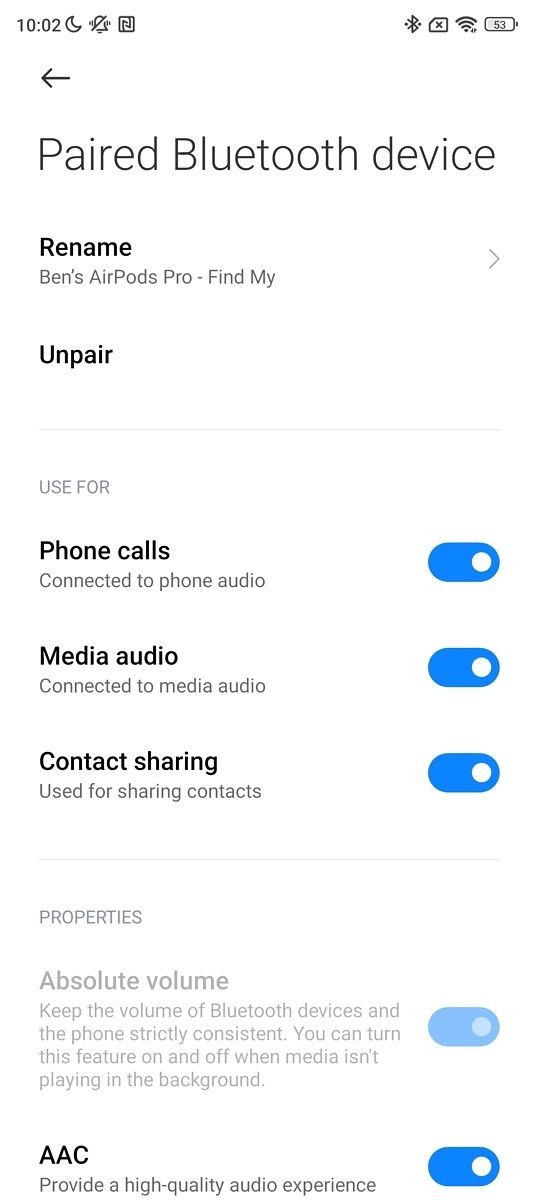The image appears to be a screenshot of a cell phone screen displaying the Bluetooth settings interface. At the top of the screen, on a black background, it indicates the time "10:02" along with a small moon icon, denoting Do Not Disturb mode. There is a diagonal line through the bell symbol, signifying that notifications are silenced. To the right, the Bluetooth symbol is visible, followed by the Wi-Fi signal icon and a battery icon showing "53," indicating 53% battery remaining.

Below, in larger black text, it reads "Paired Bluetooth device," followed by options to "Rename" the device and an entry for "Ben's AirPods Pro." This entry includes an arrow pointing to the right for further settings. In bold black text beneath, it says "Unpair," though no additional text follows this option.

Dividing lines in light gray segment the interface. The first horizontal light gray line precedes the text "Use for," also in light gray. Bold black text follows with several toggle options, each displayed with a blue elongated oval and a white dot to the right, indicating they are enabled. These options include:
- Phone calls: Connected to phone audio.
- Media audio: Connected to media audio.
- Contact sharing: Used for sharing contacts.

Another light gray horizontal line appears below. "Properties" in light gray text is listed with further options such as:
- Absolute volume: Keep the volume of Bluetooth devices and the phone strictly consistent. This is enabled, as shown by the lighter blue elongated oval.
- AAC: Provide a high-quality audio experience, also enabled with the same elongated oval and white dot to the right.

No other text is present. In summary, this screenshot details the Bluetooth settings for a cell phone, specifically configured for "Ben's AirPods Pro," showcasing various connectivity and audio settings.